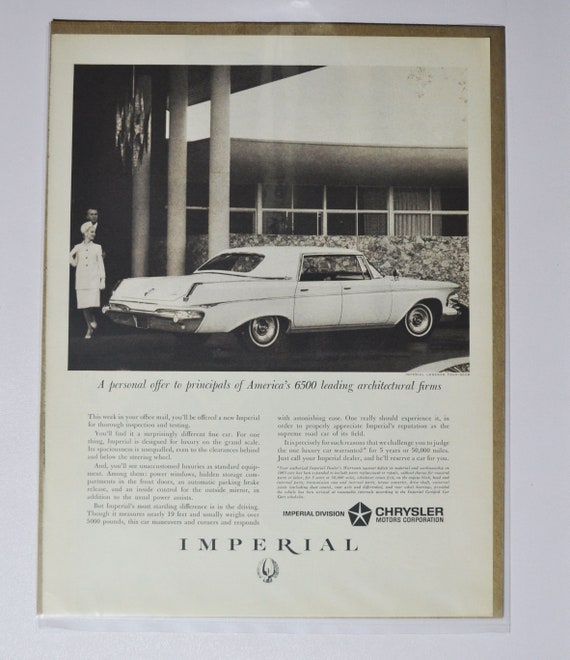This detailed image is a full-page advertisement from a 1960s magazine, presented entirely in black and white. Dominating the top half of the advertisement is a photo of a white Chrysler Imperial, a four-door car typical of the 1960s with thin white sidewalls on the tires. Both right-side windows of the car are down, revealing part of the car's sleek interior. To the left of the car are two individuals: a woman in a knee-high white dress, walking behind the vehicle, and a man standing near her, both dressed in elegant evening attire reflecting the era. Behind the car, a structure with 16 square-shaped windows, some adorned with curtains, adds an architectural backdrop. The ad features a bold headline under the photo: "A Personal Offer to Principals of America's 6,500 Leading Architectural Firms." Below this, two columns of small black text elaborate on the offer, concluding with "Imperial Division Chrysler Motors Corporation" at the bottom right of the right column. The word "Imperial" is prominently displayed across the bottom center, accompanied by a symmetrical, winged bird-like symbol with upward-curved wings. The entire composition captures a classic, sophisticated snapshot of 1960s automotive elegance and architectural prestige.